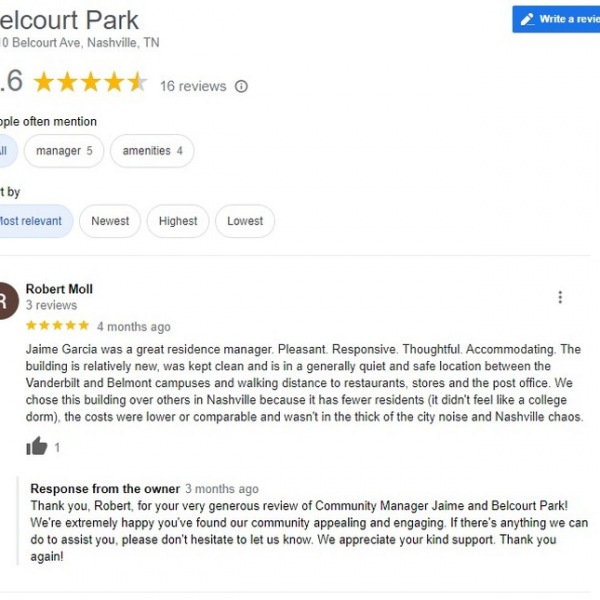**Caption:**

The screenshot showcases the "Elkhart Park" review page. At the top left, "Elkhart Park" is prominently displayed in large black text. Adjacent to this, there is a blue button with white text that says "Write a Review," although the word "review" is partially cut off. The service has received an overall rating of 4.6 stars, but the number 4 is slightly cropped off. It has accumulated 16 reviews.

Further to the left, there are buttons labeled "Manager" and "Amenities," indicating 5 reviews for the manager and 4 for amenities, respectively. Below these buttons, there are sorting options such as "Newest," "Highest," and "Lowest."

One of the reviews is highlighted below these filters. Robert Moll, who reviewed the service four months ago, gave it 5 stars. He praised Jamie Garcia, the residence manager, as being pleasant, responsive, thoughtful, and accommodating. He further mentioned that the building is relatively new, well-maintained, and situated in a quiet and safe location between the Vanderbilt and Belmont campuses, within walking distance to restaurants, stores, and the post office. Robert particularly appreciated that the building had fewer residents and did not have the feel of a college dorm, had lower or comparable costs, and was away from the city noise and chaos. His review received a thumbs up and the owner responded, thanking Robert for his feedback.